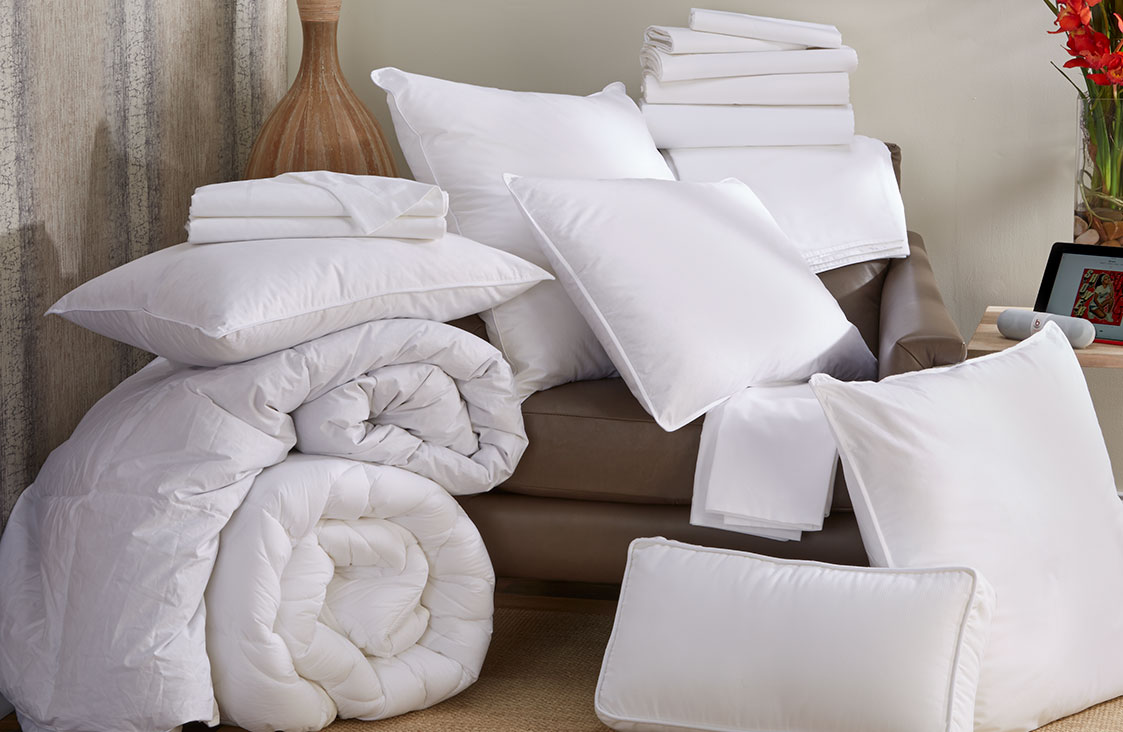The full-color photograph, clearly staged indoors under artificial light, captures a meticulously arranged setting emphasizing various white linens and pillows. The image is essentially square, though it lacks a definitive border or specific background. Central to the composition is a brown leather chair, heavily adorned with white linens: two pillows sit on the seat, another pillow leans against the right side, and several sheets are stacked on the chair's back. Directly in front of the chair, two large white blankets are rolled up on the floor, with an additional pillow resting on top of them.

To the lower right corner of the scene, more pillows and sheets are piled up on the floor, continuing the all-white theme. In the upper right corner, a glass vase containing vibrant red flowers adds a splash of color. Below this vase, a framed picture sits atop a table. The background features a light gray wall accented by a section of old wooden slabs with visible cracks on the left side, blended with a vertically patterned brown wallpaper that includes white bands.

Additionally, to the top left-center area, a wooden vase stands out against the brown wooden wall backdrop, adding a natural element to the otherwise predominantly white and brown interior scene.